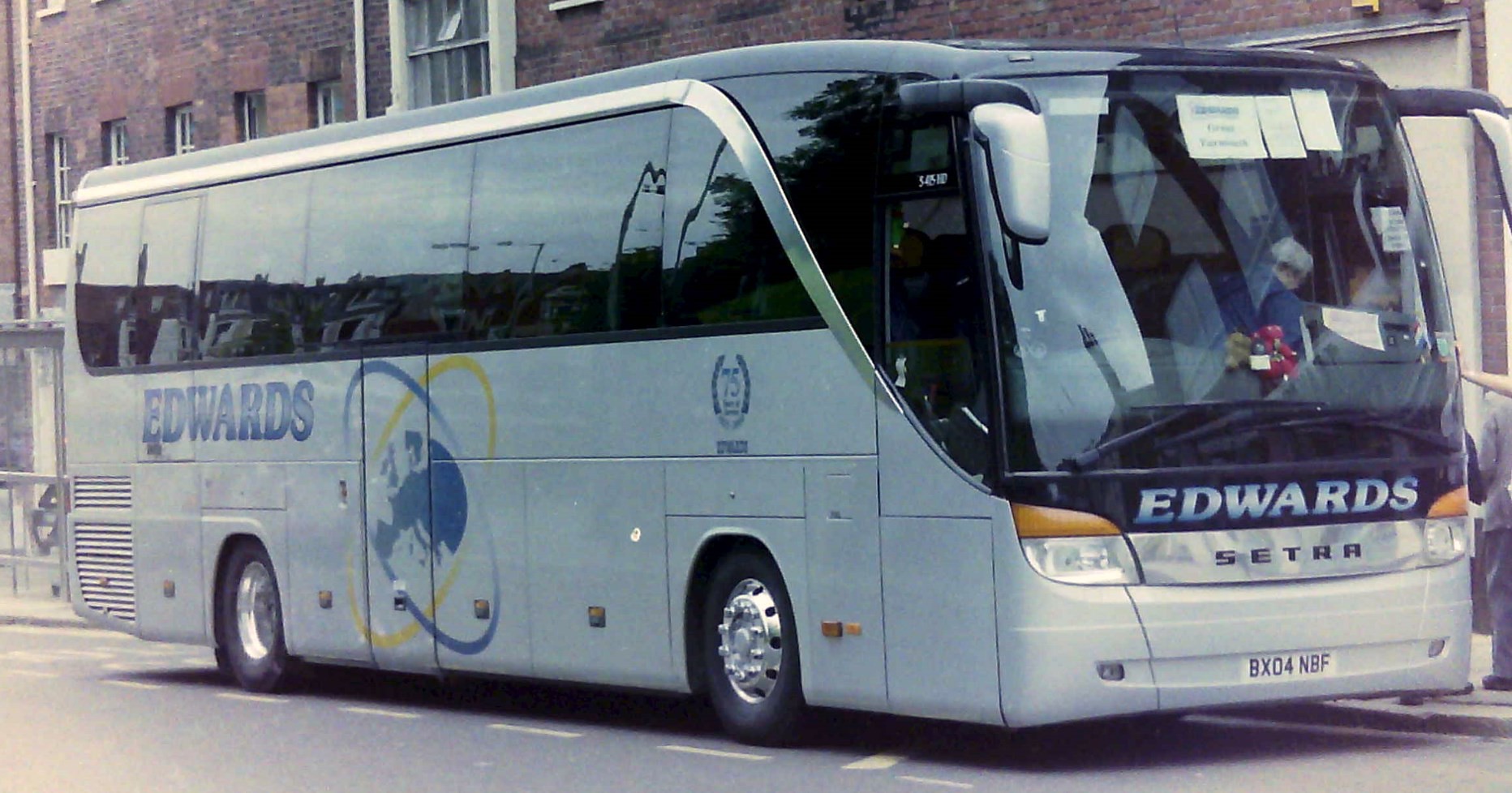This photo, taken outdoors, captures a large white bus with very dark, almost tan windows. Prominently displayed on its side is the name "Edwards," accompanied by a logo featuring a globe with one blue and one yellow circle around it. The bus is currently parked near a red brick building. In the front of the bus, a bus driver can be seen, turned halfway towards the exit instead of facing forward. The front of the bus, visible from a side angle, reveals a large window that offers a glimpse of the interior, with "Edwards" written below it, just above a number plate labeled "BX04NBF." The intricate details of the bus and its surroundings indicate that it is stationary and not in motion.